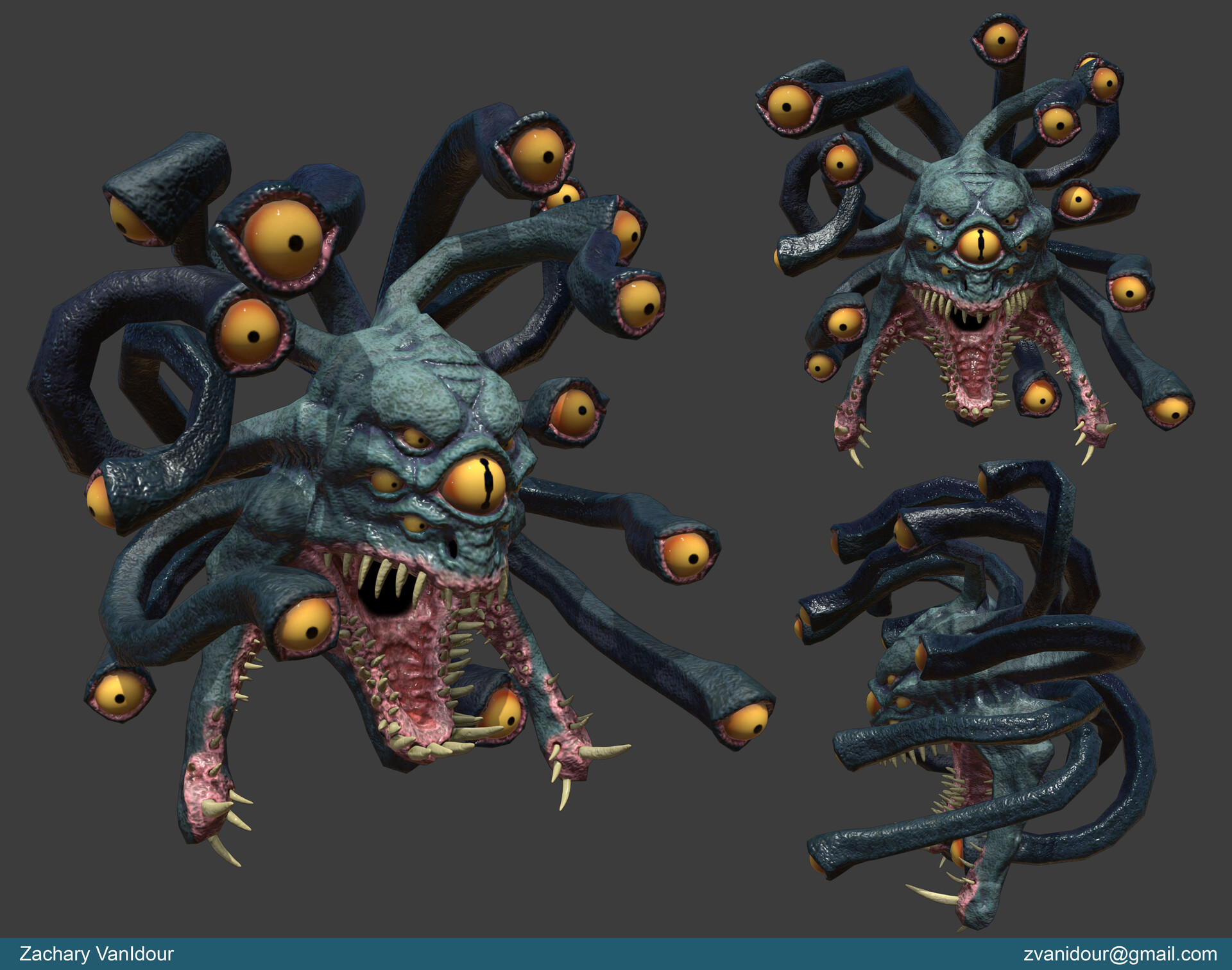The image showcases a highly detailed, computer-generated art piece of a science fiction-inspired monster, akin to a Dungeons and Dragons Beholder, created by artist Zachary Vanadour. This monstrous head features a central large eye surrounded by six smaller eyes embedded in its skull, and about a dozen tentacular stalks emanating from the back, each ending in an eyeball that can move independently. The monster's skin exhibits a gradient from light blue to dark blue, with the eyeballs displaying red to orange hues and black pupils. The open mouth, with its pinkish-red tones, is lined with many rows of drab white teeth, and additional mandibles on either side of the head also bristle with teeth or spikes. The image depicts the creature from three angles: one head gazing straight at the viewer, another at a 45-degree angle, and a third turned 90 degrees to the left, all set against a grey background. The composition emphasizes the intricate detailing of the monstrous features, especially the rows of teeth and the contrasting colors. At the bottom of the image, the artist's name, Zachary Vanadour, and his email address, zvanadour@gmail.com, are displayed.